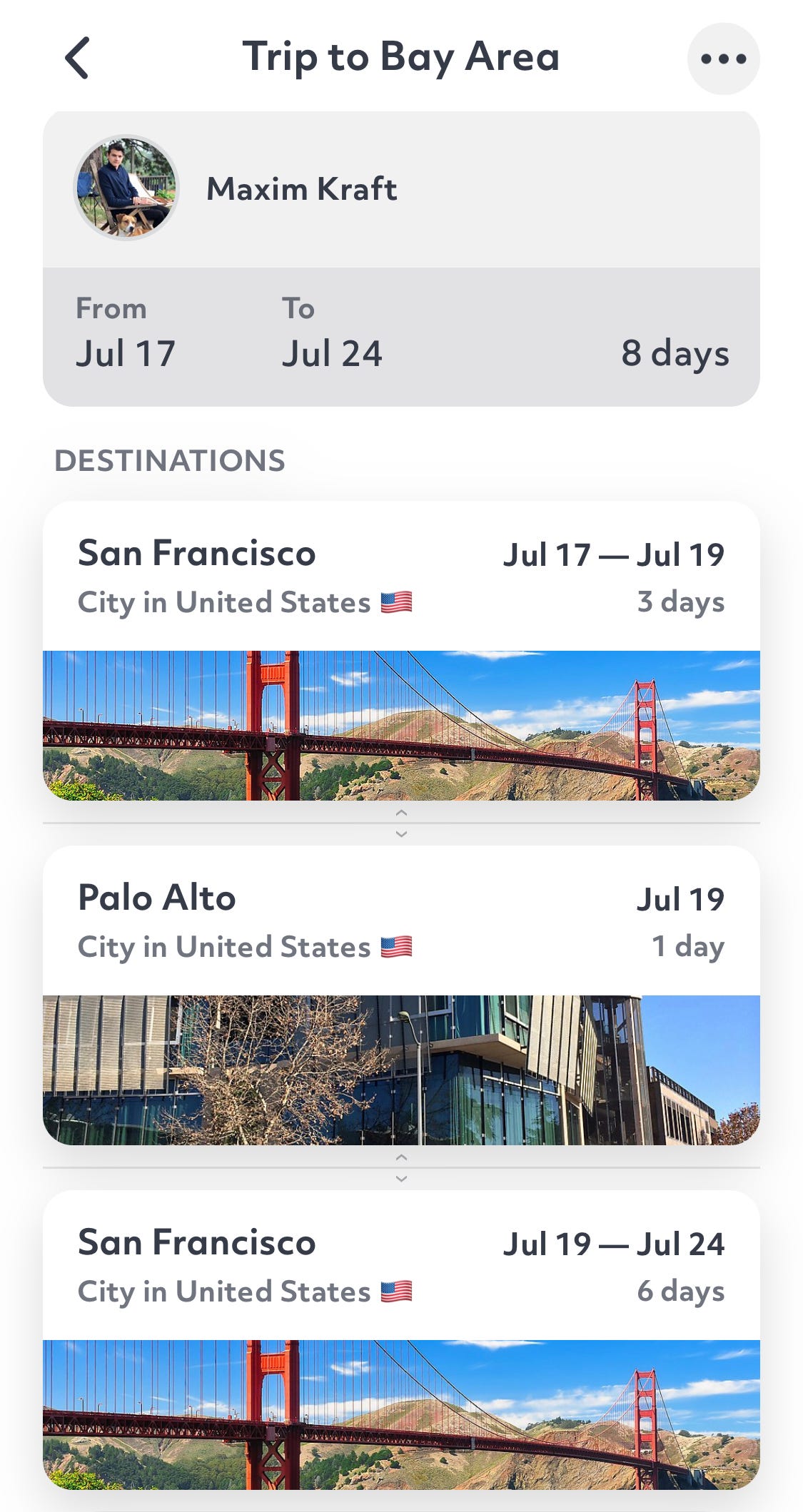Screenshot of travel itinerary posted by Maxim Kraft

The image is a screenshot of a travel itinerary shared by a user named Maxim Kraft. The user's name, "Maxim Kraft," is displayed in black font on a light gray background, accompanied by their icon. Below this, a dark gray rectangle outlines the trip duration, stating: "From July 17th to July 24th, eight days."

The itinerary features three destinations listed in rounded rectangular sections. Each section includes details and an image:

1. **San Francisco (July 17th - 19th)**
   - **City:** United States
   - **Days:** 3
   - **Flag:** U.S. flag icon
   - **Image:** A picture of the iconic Golden Gate Bridge

2. **Palo Alto (July 19th)**
   - **City:** United States
   - **Days:** 1

3. **San Francisco (July 19th - 24th)**
   - **City:** United States
   - **Days:** 6
   - **Flag:** U.S. flag icon
   - **Image:** Another picture of the Golden Gate Bridge